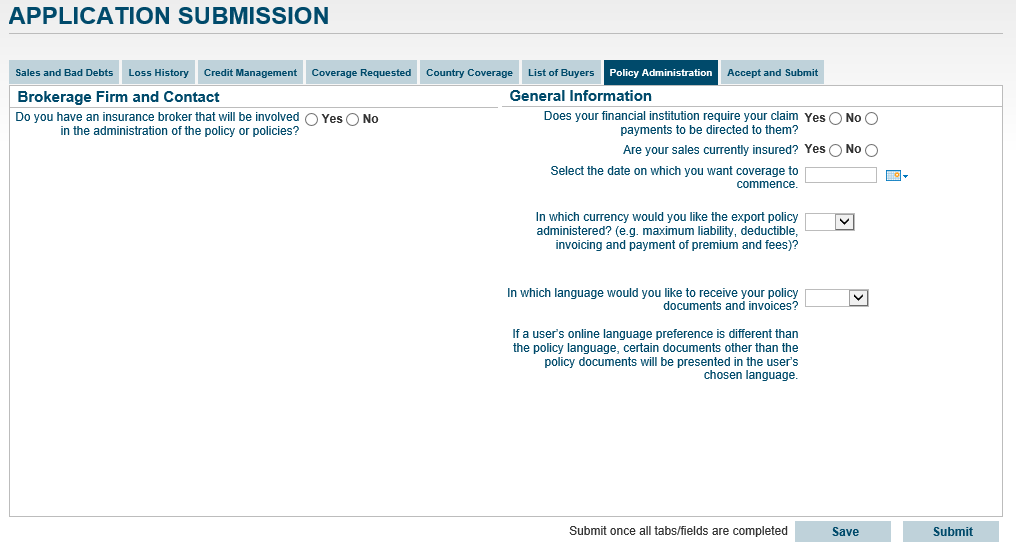This image captures an application submission interface in the process of being completed. At the top left, the header "Application Submission" is prominently displayed in blue writing. Below this, a series of tabs are presented, each with a blue background and dark blue text, labeled as follows: Sales and Bad Debts, Loss History, Credit Management, Coverage Requests, Country Coverage, List of Buyers, Policy Administration, Accept and Submit, and Brokerage Firm in Contact. 

On the right side of the interface, you have a section titled "General Information." Here, users are asked whether they have an insurance broker involved in the administration of the policy. There are options for "Yes" and "No." Another question asks if their financial institution requires the claim, with "Yes" or "No" options available. Following this, users are asked if their financial institution requires claim payments to be directed to them, and if their sales are currently insured, both with "Yes" or "No" options.

Users are also prompted to select the date they want the coverage to commence through a designated date-selection box. They must specify in which currency they would like to handle policy administration, maximum liability deductible, invoicing and payment, or premiums and fees, with a clarifying question mark in parentheses. Additionally, they are asked in which language they would prefer to receive their policy documents and invoices. A note clarifies that if a user's online language preference differs from the policy language, certain documents other than the policy documents will be presented in the user's chosen language.

At the very bottom of the interface, users are prompted to submit the form once all tabs and fields are completed, with both "Save" and "Submit" buttons available.